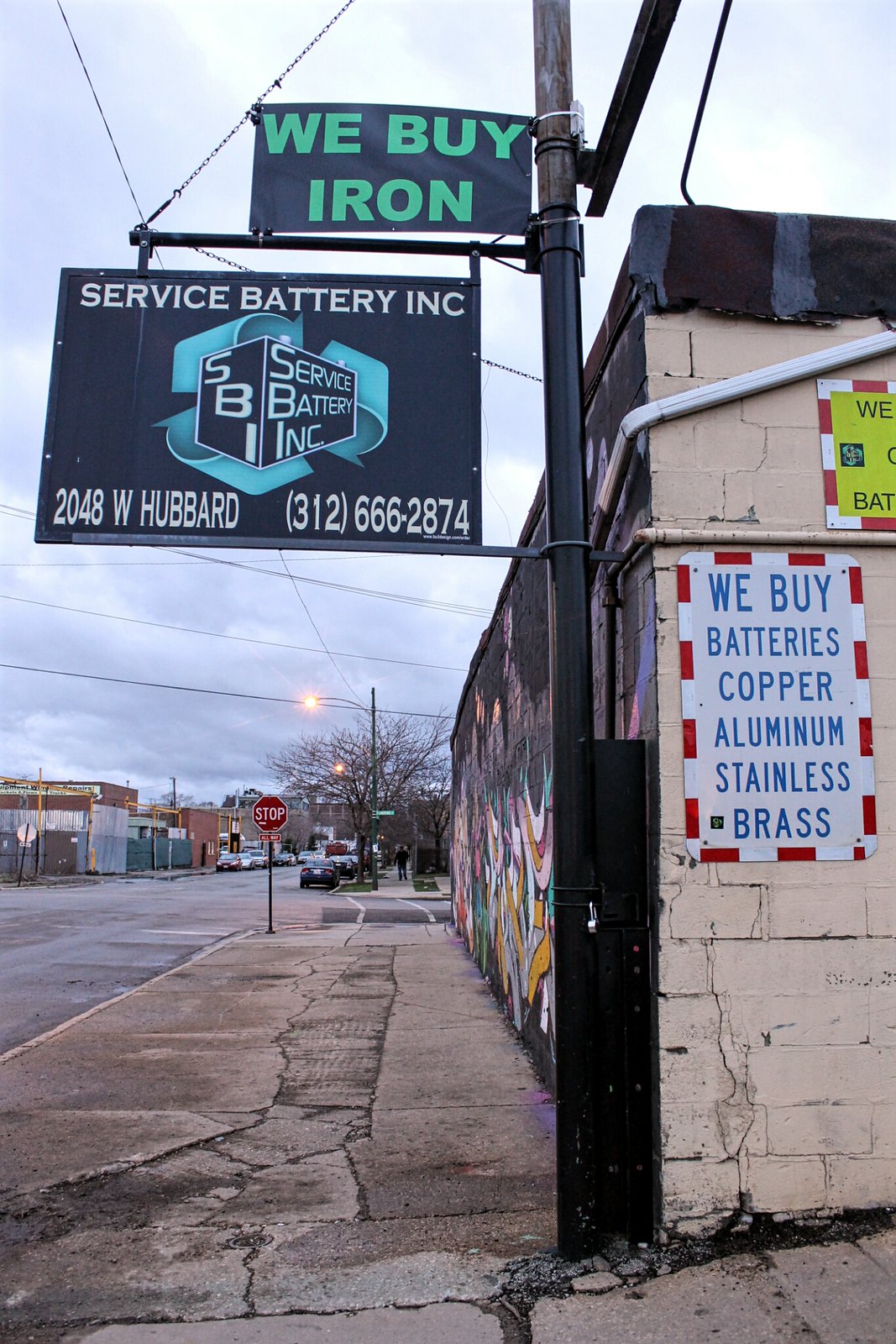The photo captures an urban street scene dominated by a beige brick building at the corner. A black pole prominently stands near the corner, with multiple signs affixed to it. The highest sign, in green letters on a black background, reads "We Buy Iron." Below it, a more substantial sign for "Service Battery Inc." features a blue recycling arrow design and provides the address, "2048 West Hubbard," and the phone number "312-666-2874" in white text. Alongside the pole, the building’s façade displays a white sign advertising "We Buy Batteries, Copper, Aluminum, Stainless, Brass." The street unfolds into the distance with a stop sign visible down the road. The sidewalk, paved with somewhat dirty beige stone, borders an empty road with low-profile buildings and a dead tree ahead. The sky is overcast, filled with dark, gray clouds.